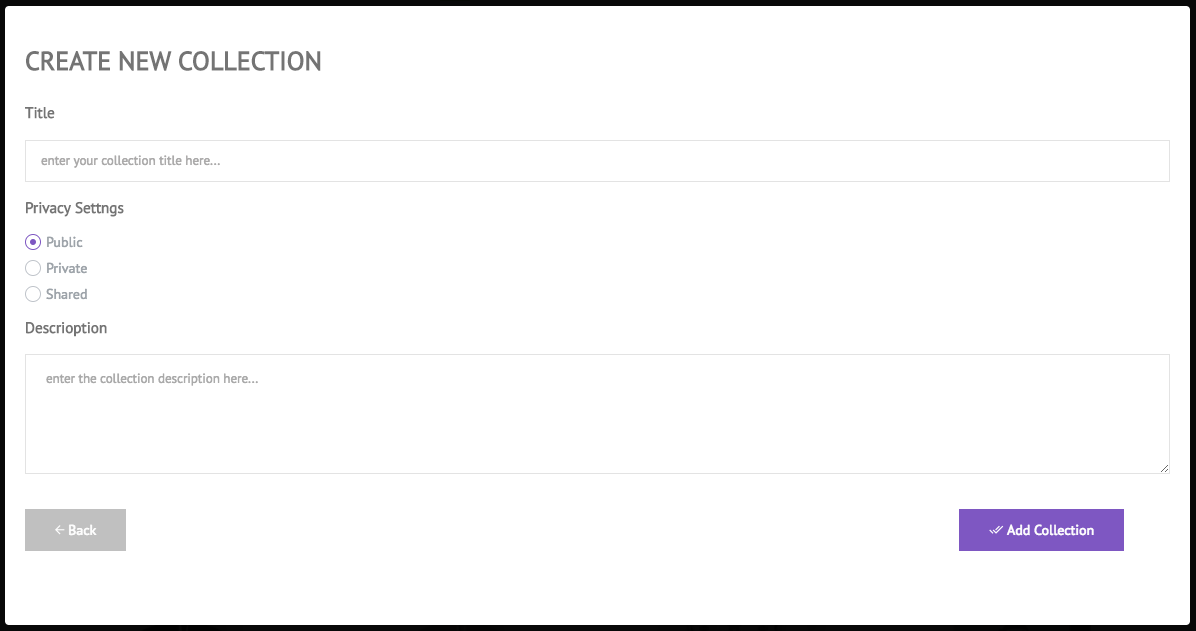**Caption: Interface of a New Collection Creation Page**

The image displays the user interface for creating a new collection on a website. At the top left, there is a section with black text that serves as the title. Below it, a placeholder text reads "Enter your collection title here." The privacy settings options are located next, with checkboxes for "Public," "Private," and "Share" - all currently unchecked. A description field with the placeholder text "Enter the collection description here" is present, and a grey rectangular button labeled "Back" is positioned nearby. The "Add Collection" button is prominently shown in purple.

The rest of the interface is mostly white with minimal visual elements. The central portion of the window reiterates options for adding a title to the collection, privacy settings with "Public," "Private," and "Share" choices, and a general collection setup for the website. The layout is bordered with clean edges and an overall simple, functional design.